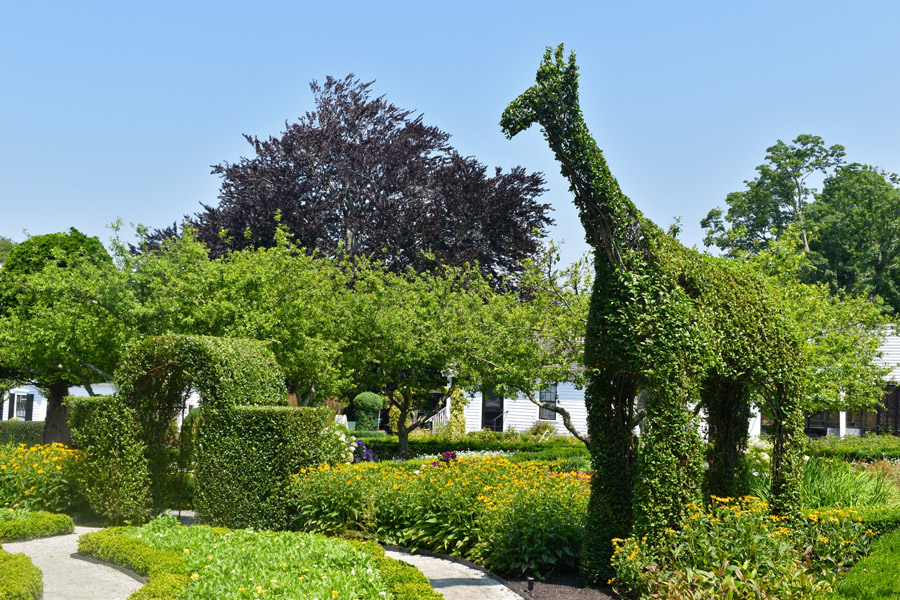The image depicts a vibrant garden scene dominated by meticulously trimmed hedges. At the forefront stands a towering hedge sculpted into the shape of a giraffe, showcasing impressive topiary skills. To the left of the giraffe hedge, a curving walking path leads to an intricately carved archway, also fashioned from lush greenery. The garden is populated with a variety of plants, including clusters of yellow-orange flowers and neighboring Lazy Susan blooms, adding bursts of color amidst the sea of green. Tall trees, including a striking tree with red leaves and another with dark, purple-black foliage, provide a dramatic backdrop. In the distance, partially obscured by the dense greenery, stands a white house, hinting that this artistic garden is part of a residential neighborhood. The clear blue sky overhead completes the picturesque, sunny day scene.